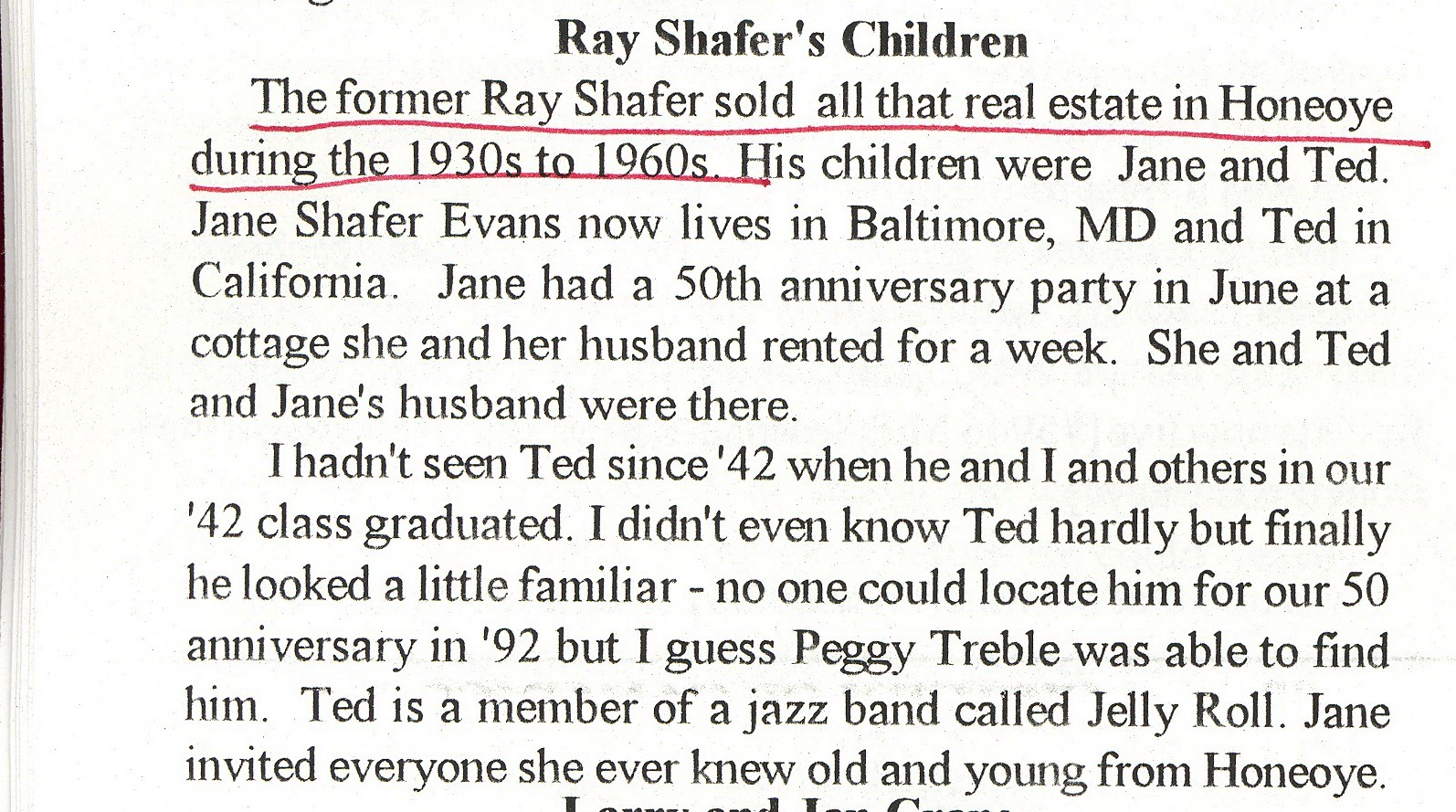The image is an excerpt from a book or magazine, featuring a white background with visible edges of the scanned or photographed page on the left. At the top center of the page, a bold black title reads "Ray Schaefer's Children." Below the title, the first sentence is underlined in red and in non-bold black font. It reads, "The former Ray Schaefer sold all that real estate in Hanoi during the 1930s to 1960s." The text continues to detail that his children, Jane and Ted, now live in different states, with Jane Schaefer Evans residing in Baltimore, Maryland, and Ted in California. Jane celebrated her 50th anniversary in June at a rented cottage, attended by herself, Ted, and her husband. The narrator mentions not having seen Ted since their class of '42 graduation and barely recognizing him. Ted, a member of a jazz band called Jelly Roll, was eventually located by someone named Peggy Treble for a 1992 reunion. Jane invited everyone she knew from Hanoi to her anniversary event.